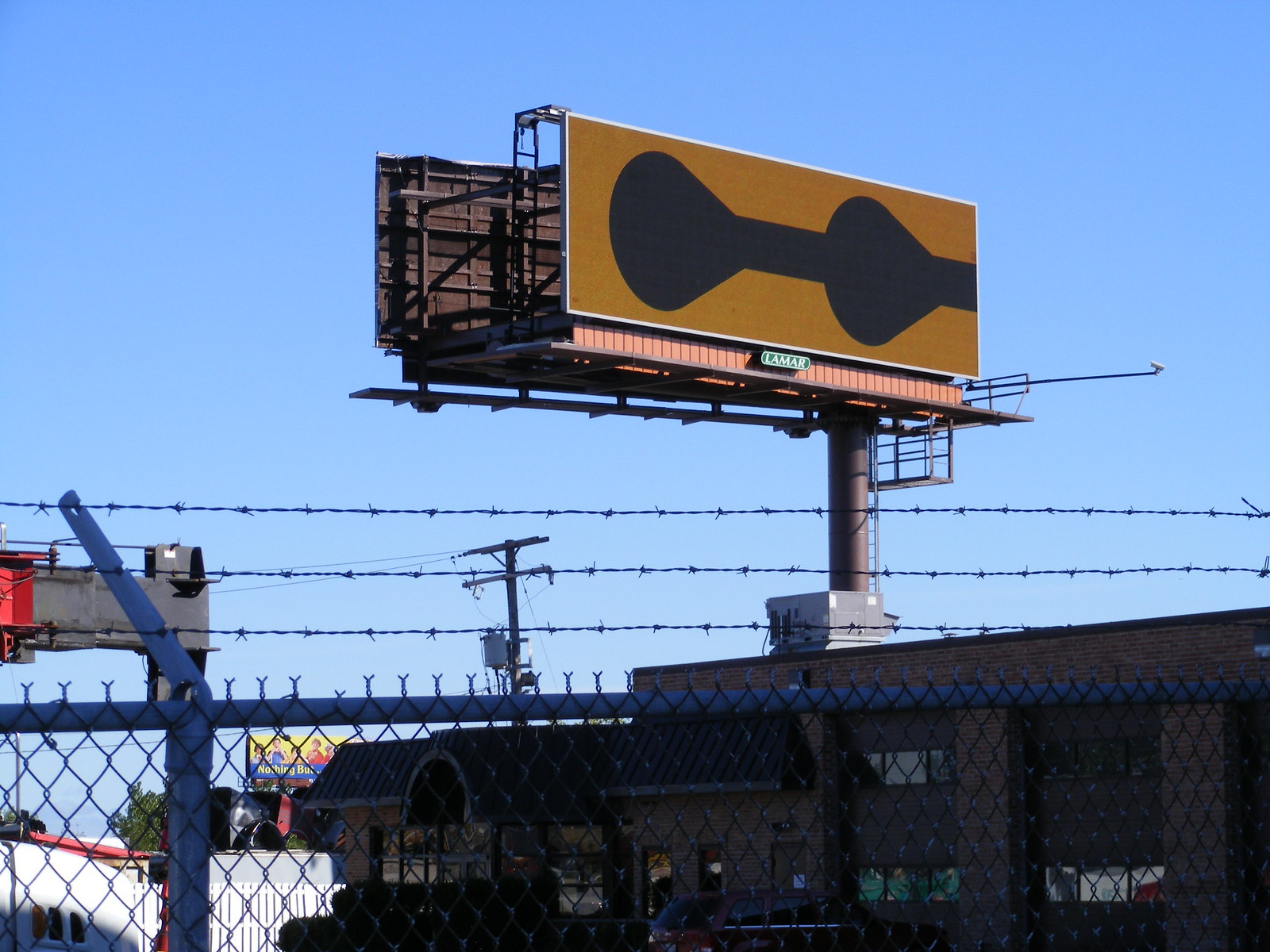This photograph captures a scene through a silver-colored chain-link fence topped with three rows of barbed wire. In the foreground, the fence stretches across the width of the image, emphasizing the barrier between the viewer and the background. Behind the fence, a two-story warehouse-like building occupies about two-thirds of the bottom half of the image. This building features large garage doors on the right side and an awning on the left, indicative of a commercial or small business space.

In the middle to background, a large, two-sided billboard stands prominently on a post with its base appearing to be red and supported by a silver-colored cylindrical structure. The billboard's sign, outlined in white, has a distinct yellow to goldish-brown background, showcasing two black shapes that resemble stacked hourglasses or chemistry beakers placed atop one another. Notably, there is no writing on the billboard. Above this main building, another billboard's edge is faintly visible, complementing the clear light blue sky overhead. Power lines are also discernible in the background, adding to the industrial ambiance of the scene.